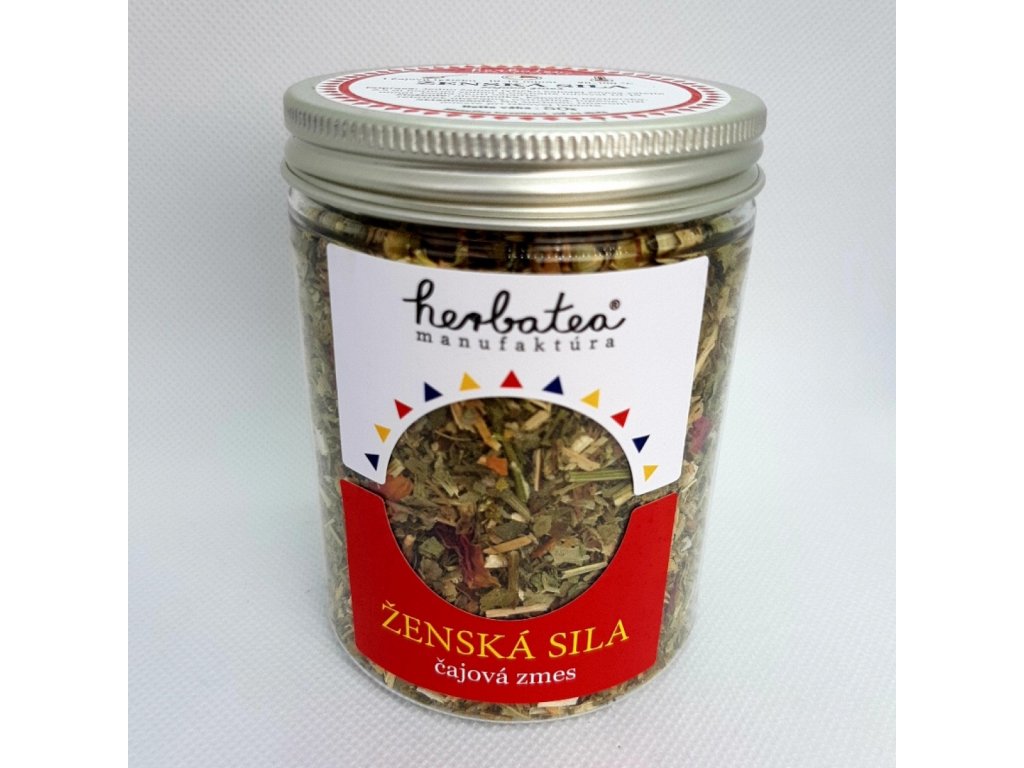This close-up photograph, set against a stark white background, features an unopened glass jar of herbal tea, identified as "Herba Tea." The jar, standing upright, has a silver lid and sports two distinct labels. The top label is white with multi-colored triangles in blue, yellow, and orange, while the bottom label is a vibrant red with yellow text reading "Herba Tea" followed by white text below that. The tea blend, referred to as "Zenska Sila" and "Katajova Zmes," suggests Eastern European origins. Through a small, unobstructed viewing window in the labels, one can see a mixture of various herbs inside the jar, showcasing shades of green, yellow, white, and beige, with hints of dried chives among the assortment. The overall presentation hints at a commercial product photo, potentially intended for a website or retail promotion.